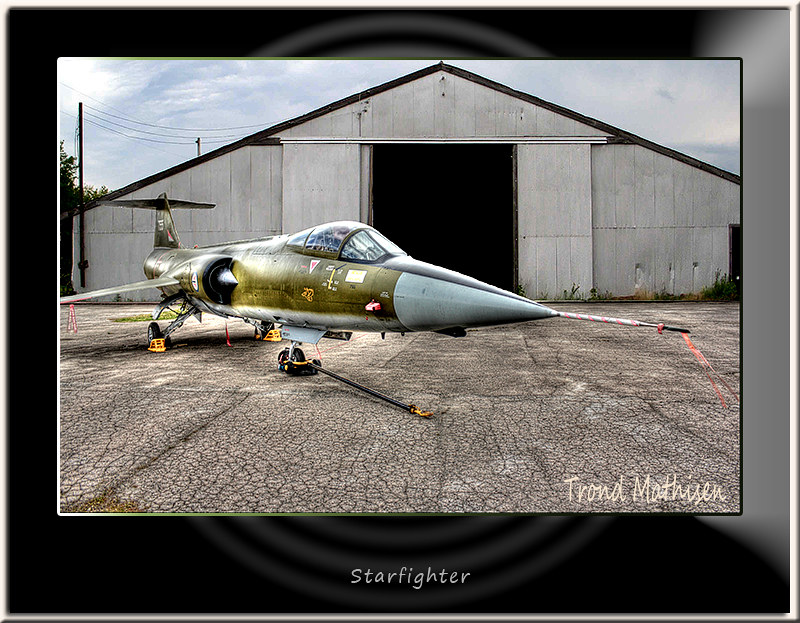This photo captures an old fighter jet from the 1960s parked on a cracked concrete surface outside what appears to be a large metal warehouse or airplane hangar. The warehouse, otherwise gray and nondescript, has its sliding doors open, revealing a pitch-black interior. The jet features a sleek design with a long, silver-tipped nose cone and an otherwise army green and brown paint job. It appears small in comparison to modern-day fighter planes and sports yellow blocks around its wheels, preventing it from rolling. Additionally, a jack-like apparatus with a handle is attached to the front wheel, indicating it can be manually maneuvered. Detailed markings, including a small sword design on the side, adorn the aircraft. This classic fighter jet, likely intended for a single pilot, is labeled "Starfighter" in text printed beneath the image, which credits Tron Matherson as the photographer.